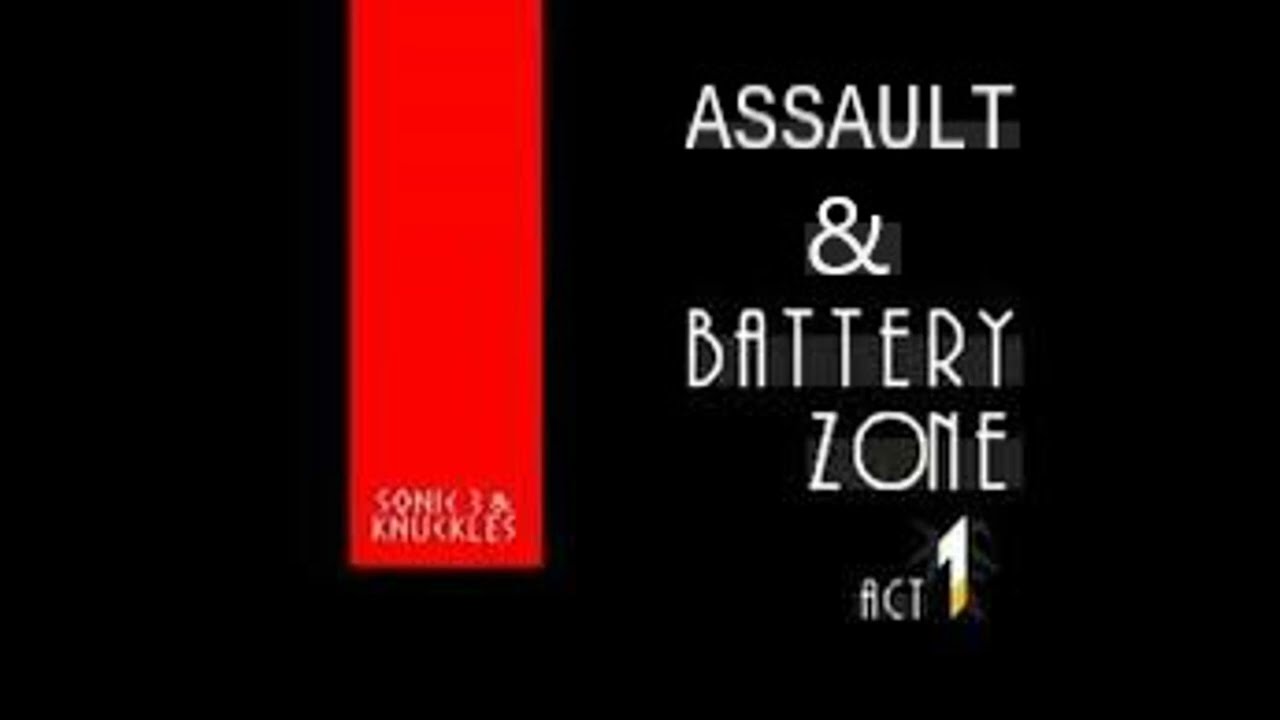The image features a stark black background with prominent white text slightly right of center at the top. This white text, all in capital letters, reads "ASSAULT & BATTERY ZONE ACT 1," with each word stacked vertically. The word "ACT" is smaller in print compared to "BATTERY," "ZONE," and "ASSAULT." Beneath the word "ACT," the number "1" appears, larger and thicker than the other letters, with a subtle, ghostly gold hue towards its base.

To the left of the text, a red banner hangs down almost three-quarters of the way from the top. This banner features faint, blurry white letters at its bottom, spelling "SONIC" followed by "KNUCKLES," both of which are partly obscured by red bleeding into the text, rendering it fuzzy. The banner is lined by faint vertical bars that run down its left and right sides, stopping just above the bottom text.